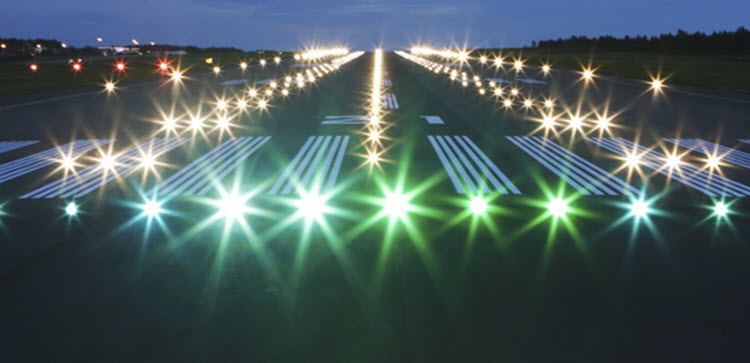This is a detailed night-time photograph of an airport runway, dramatically lit up with various colored lights that give an almost star-like quality to the entire scene. The runway, which appears to stretch endlessly into the horizon, is flanked on both sides by a series of bright white lights that also line the middle and outer edges further down the pathway. The lights create a striking visual effect, almost as if rows of stars are paving the way. Red lights are visible on the left side of the runway, adding to the colorful illumination, though their exact purpose remains unclear.

At the forefront of the image, there's a mixture of green and bluish lights, possibly due to the camera capturing the scene in a particular way. The runway itself is marked with numerous white dashes and stripes, reminiscent of crosswalk markings, which guide where planes should land. There is grass and foliage visible towards the right side of the runway, and in the distance, there seems to be a building obscured by darkness and the glow of the lights.

The top portion of the image reveals a thin line of blue night sky, contrasting against the glittering array of lights below. The overall impression is of a meticulously organized, brightly lit runway, almost otherworldly in its luminescence and extending into the night with an infinite quality.